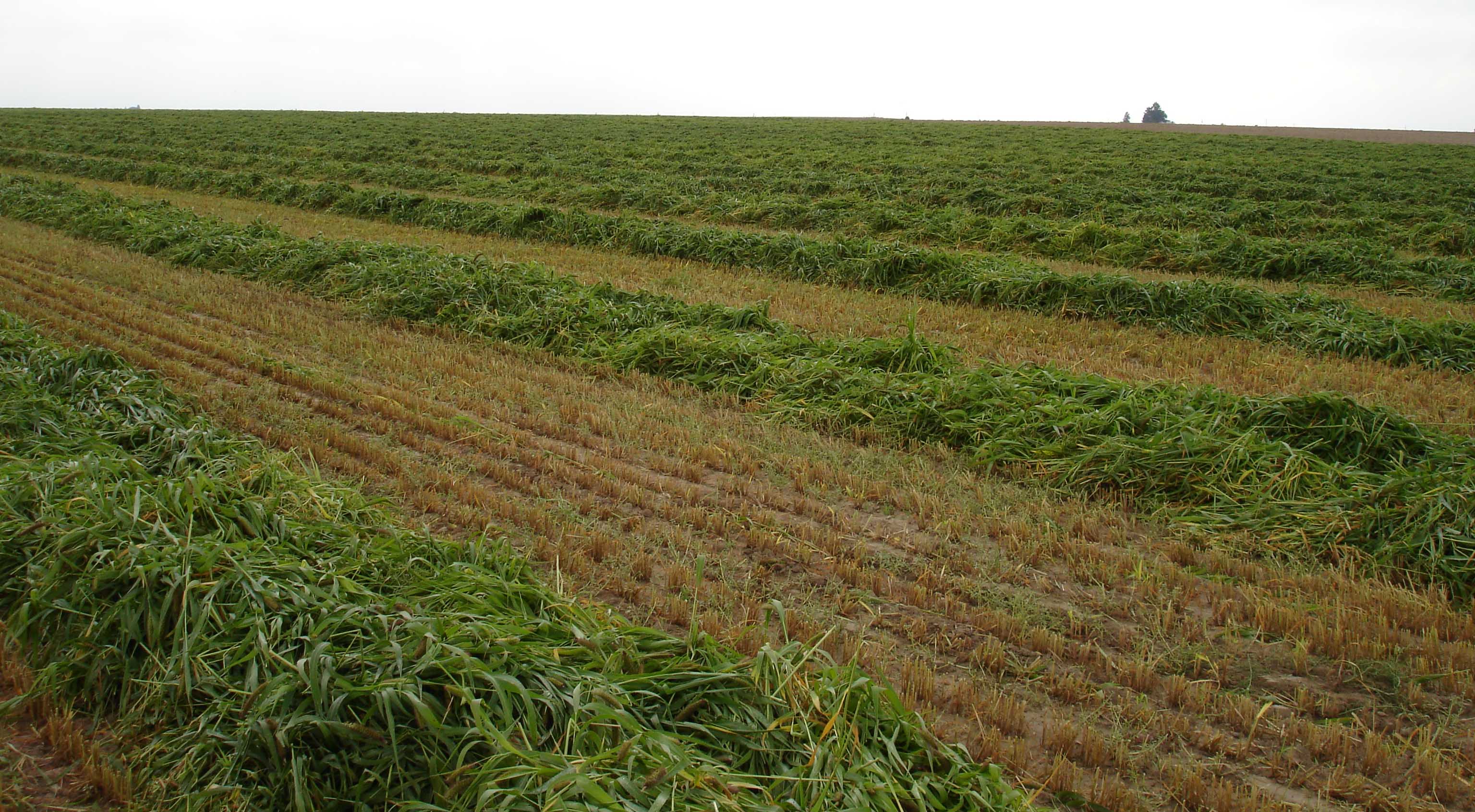The image depicts a recently harvested farmland, with rows of shorter, brownish, freshly cut grass interspersed with taller, dense, green foliage. The symmetrical lines of crops reveal a well-organized agricultural layout. At the center, these almost diagonal lines stretch across the field, highlighting the contrast between the shorter trimmed areas and the lush green rows. In the background, the sky is grayish and overcast, hinting at an early morning or late afternoon setting. On the distant top right, a building stands out against the horizon, breaking the monotony of the field. Additionally, trees are faintly visible along the horizon, adding depth to the pastoral scene.